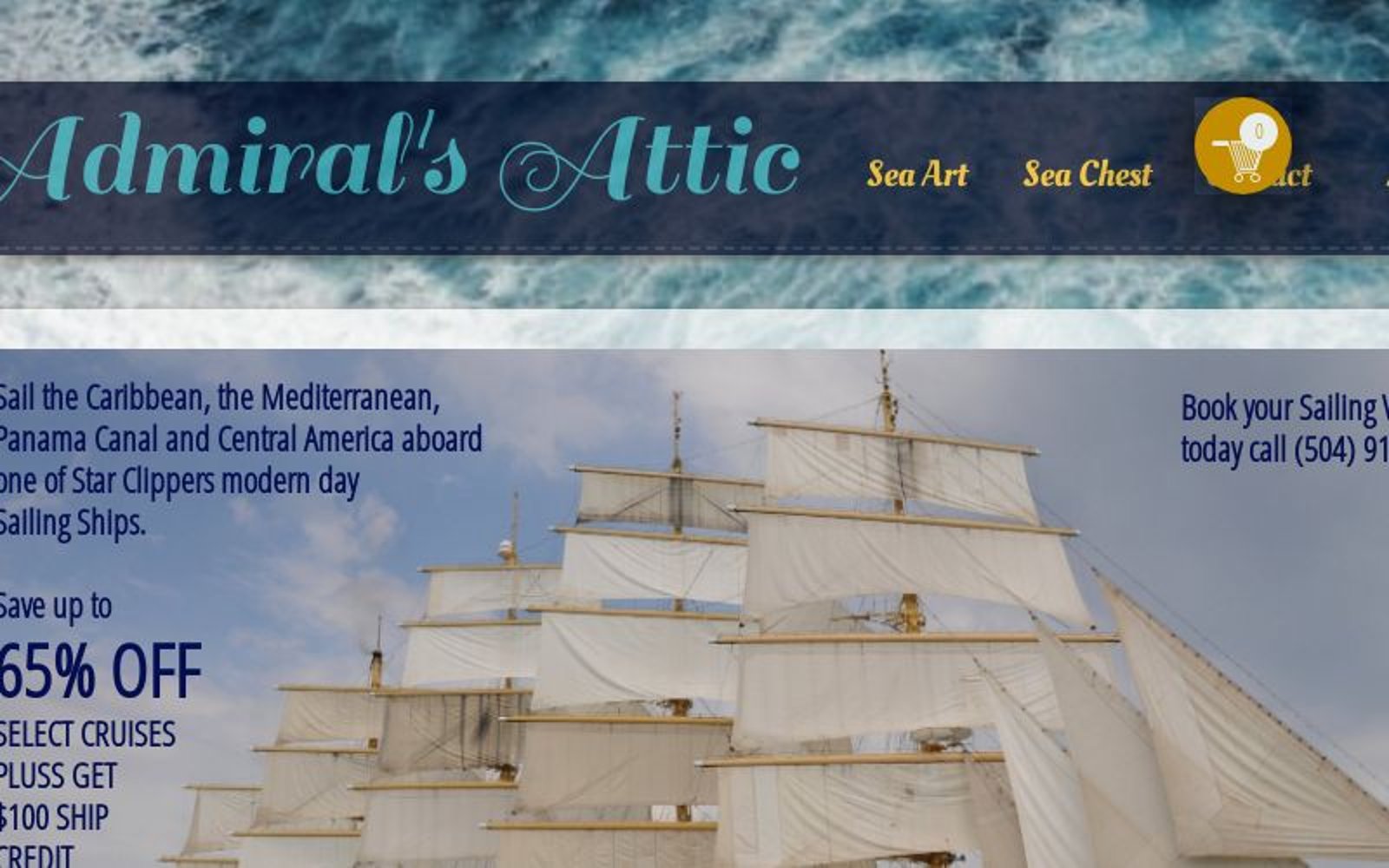The image is a detailed, landscape-oriented color photograph used for an advertisement. At the top of the image, there's a sky or ocean-themed horizontal rectangle in aqua and white hues, overlaid with a dark blue tinted rectangle. This section features the text "Admiral's Attic" in aqua script on the left, followed by "Sea Art" and "Sea Chest" in red italics. A gold circle with a white shopping cart icon indicating an online store option appears at the top right.

The photograph below this header showcases a collection of nautical-themed items arranged in a room. To the right, a framed print of a steamship cruise liner hangs on the wall with a model ship below it. Scattered throughout the room are an array of maritime artifacts: a sailor's hat atop a tripod in the center, a black and white striped lighthouse on the bottom left, a globe, and various ship lights. Also visible are a mounted gold gauge, paddles, and an oar. The scene is densely packed with sea decor trinkets, creating a rich, nautical ambiance. The overall style blends photographic realism with graphic design elements, ideal for a digital advertisement.